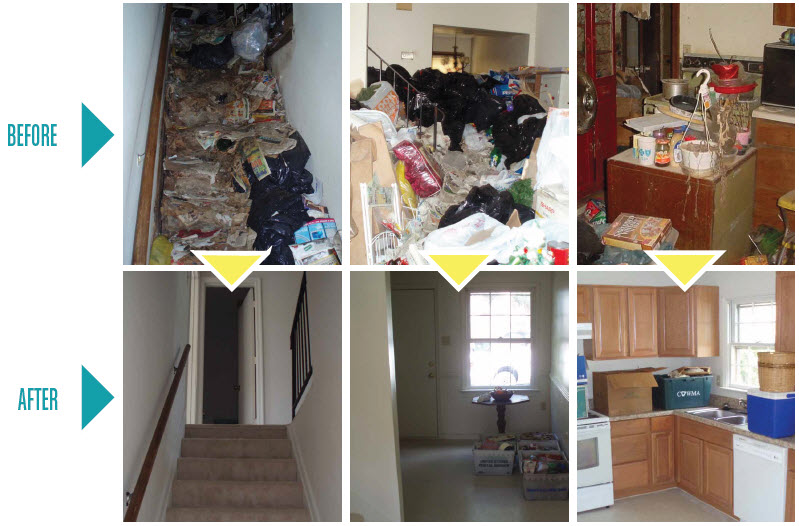The image is a rectangular collage of six full-color photographs, visually divided into a top and bottom row with a large white border surrounding the entire collage and thin white lines separating each photograph. The top row, labeled "before," consists of three images depicting various rooms of a hoarder's home in a state of extreme disarray. On the top left, a staircase is obscured by heaps of garbage, including black plastic trash bags, old newspapers, containers, magazines, comic books, and boxes, rendering it nearly impassable. The center top image reveals a room, possibly a living or dining area, filled to the brim with black trash bags, plastic containers, newspapers, and other debris, creating an almost impenetrable barrier. The top right image shows a kitchen in dilapidation, featuring a dying potted plant on the countertop, old cereal boxes, dirty dishes, and everything covered in grime, with red-painted furnishings in disrepair.

The bottom row, labeled "after," offers a contrasting view, showcasing the same areas post-cleanup. The bottom left photograph presents the staircase, now immaculate and seemingly brand new, devoid of any clutter. The center bottom image mirrors the transformation of the previously trashed room; it’s now tidy with a few belongings neatly organized in plastic boxes. The bottom right photograph reveals the kitchen, now restored with polished wooden cabinets and a completely clean and orderly space. The collage effectively demonstrates the drastic improvement from a chaotic, unlivable state to a clean, organized environment through the before-and-after photographic comparison.